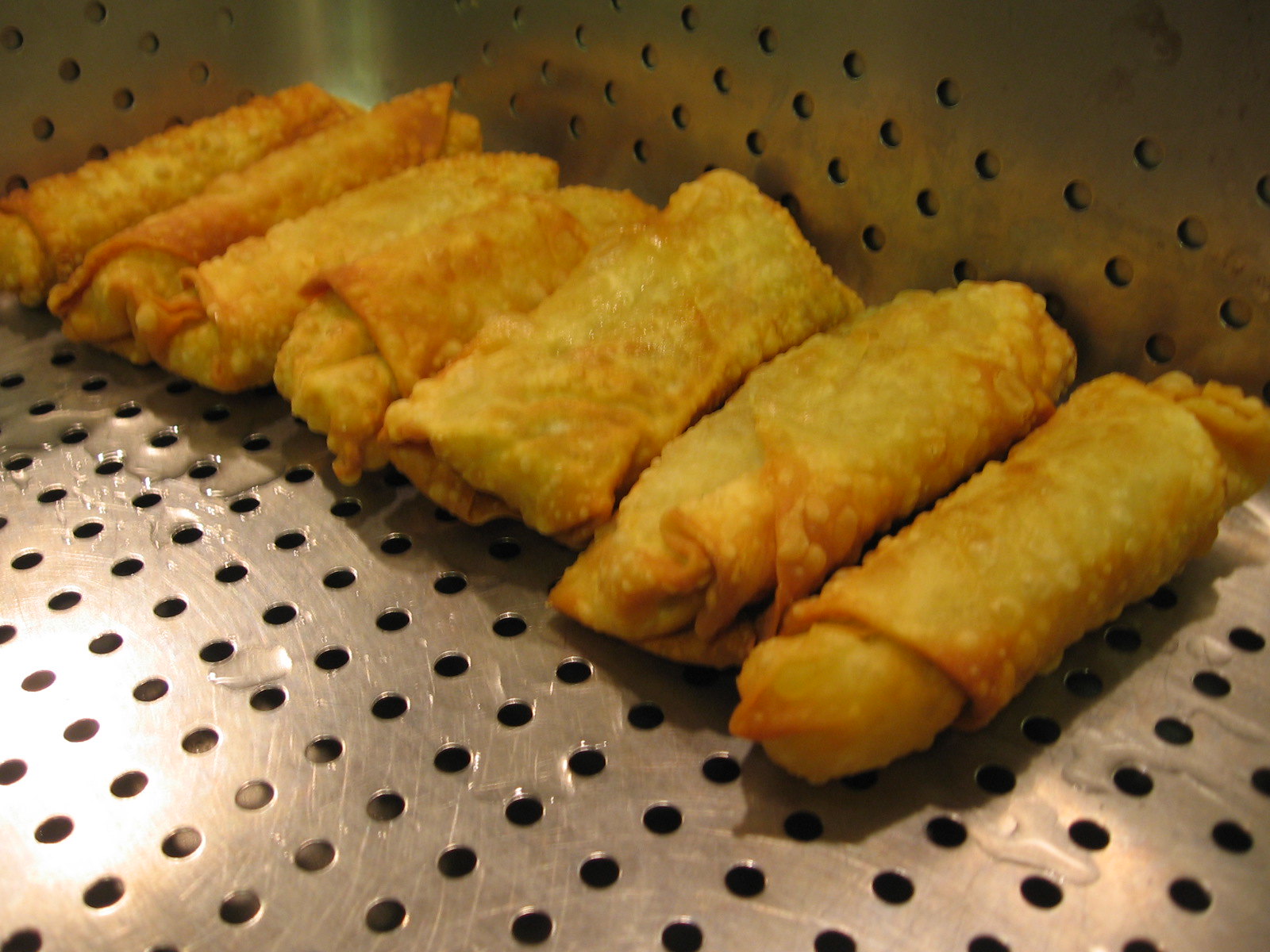The image is an amateur photograph of approximately seven golden-brown fried egg rolls, arranged diagonally across a silver metal tray with numerous holes for straining oil. The egg rolls are lined up in a single row and appear larger towards the bottom right and smaller towards the top left, indicating a slight perspective. The metal tray, possibly from a fryer, shows evidence of frying with a small puddle of liquid, likely grease or condensation, in the top left corner. The egg rolls are visibly fresh, with one in the center still glistening with oil and exhibiting crispy bubbles along its surface, particularly at the edges where the wrappers are darker golden-orange. The bottom left corner of the tray is empty, further emphasizing the metallic, perforated surface.